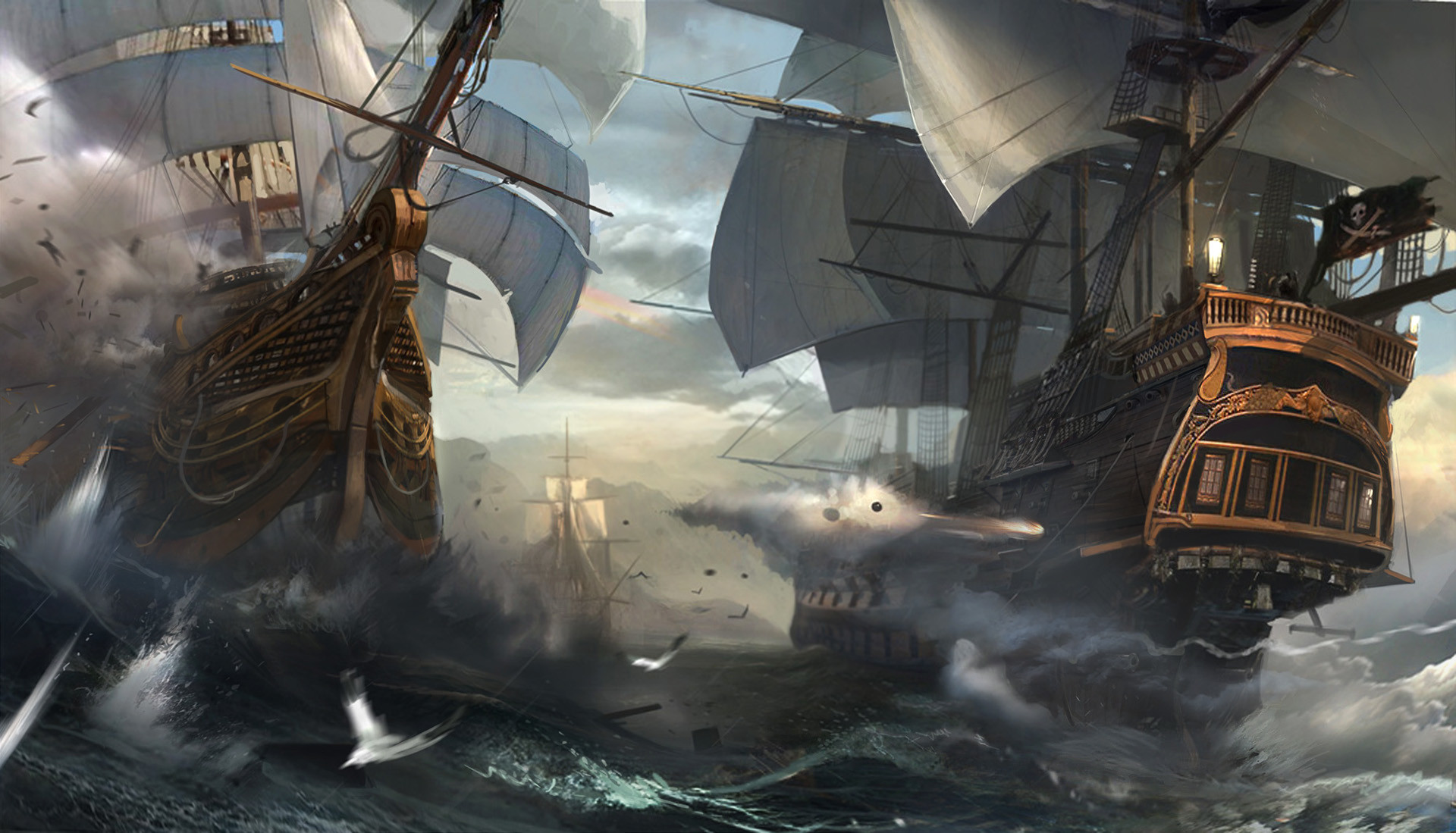The detailed drawing depicts a dramatic scene of a storm at sea where three wooden ships with white masts and sails are caught in turbulent waters. The dark, stormy sky looms overhead, reflecting the severity of the situation. The sea is rough, with white-capped waves crashing fiercely against the vessels. Two prominent ships dominate the foreground. The ship on the right, with a sharp pointy prow adorned with intricate patterns, appears to be engaging the ship on the left, evidenced by the cannon fire and resulting damage. This ship has five windows on its flat front, above which sits a curved decorative piece. The second ship, also crafted of wood and with noticeable fancy carvings, shares the same traditional, old-world construction, suggesting a historical setting possibly reminiscent of early world battles. In the backdrop, a third ship adds depth to the chaotic scene, underscoring the extensive turmoil wrought by the storm and conflict.